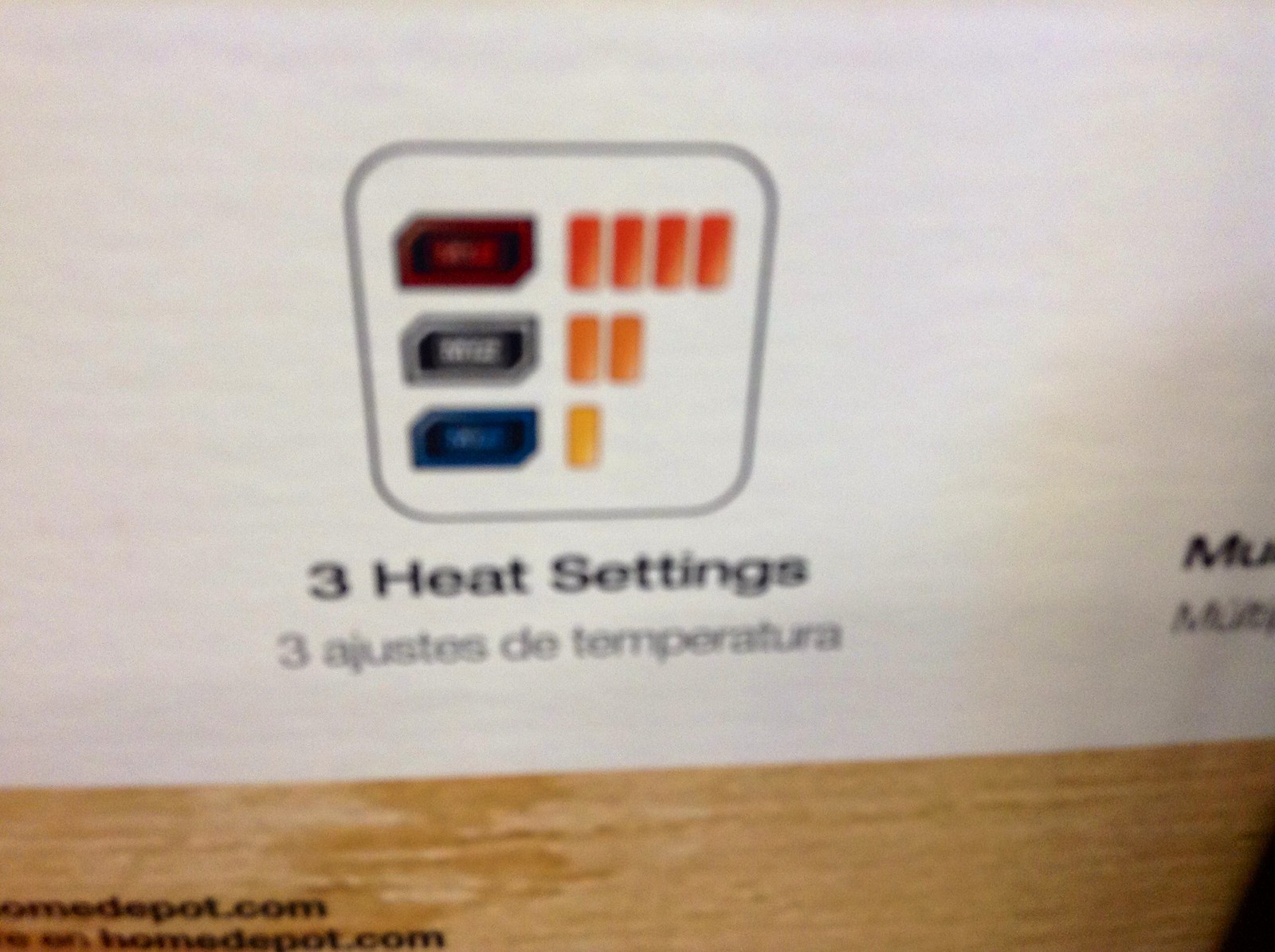Image Caption: A white instruction paper, possibly included with a product purchase, occupies the center of the image. This paper, which appears to be made of standard white material, features a decorative wood-grain border at the bottom. Dominating the center of the paper is a black square with rounded edges, containing a complex diagram.

Within this black square, there is a prominent red rectangle with a black border, displaying text in red. Adjacent to this red rectangle are four orange rectangular bars that resemble batteries. Below the red rectangle is a white rectangle with black sides, white text, and a white outline, accompanied by two more orange rectangular bars on its right.

Further below, a black rectangle with a blue outline displays text in blue; next to this rectangle is a single orange rectangular bar. Directly beneath this central black square, large bold black letters read "Three Heat Settings," followed by a smaller, italicized translation in Spanish: "Tres ajustes de temperatura."

On the right edge of the paper, the partial word "MU" is visible in bold letters, partially cut off and appearing alongside blurry, partially visible Spanish text. The bottom of the document is dominated by the wood-grain border, within which the text "homedepot.com" is printed in black font, immediately followed by the phrase "en homedepot.com" just below it.